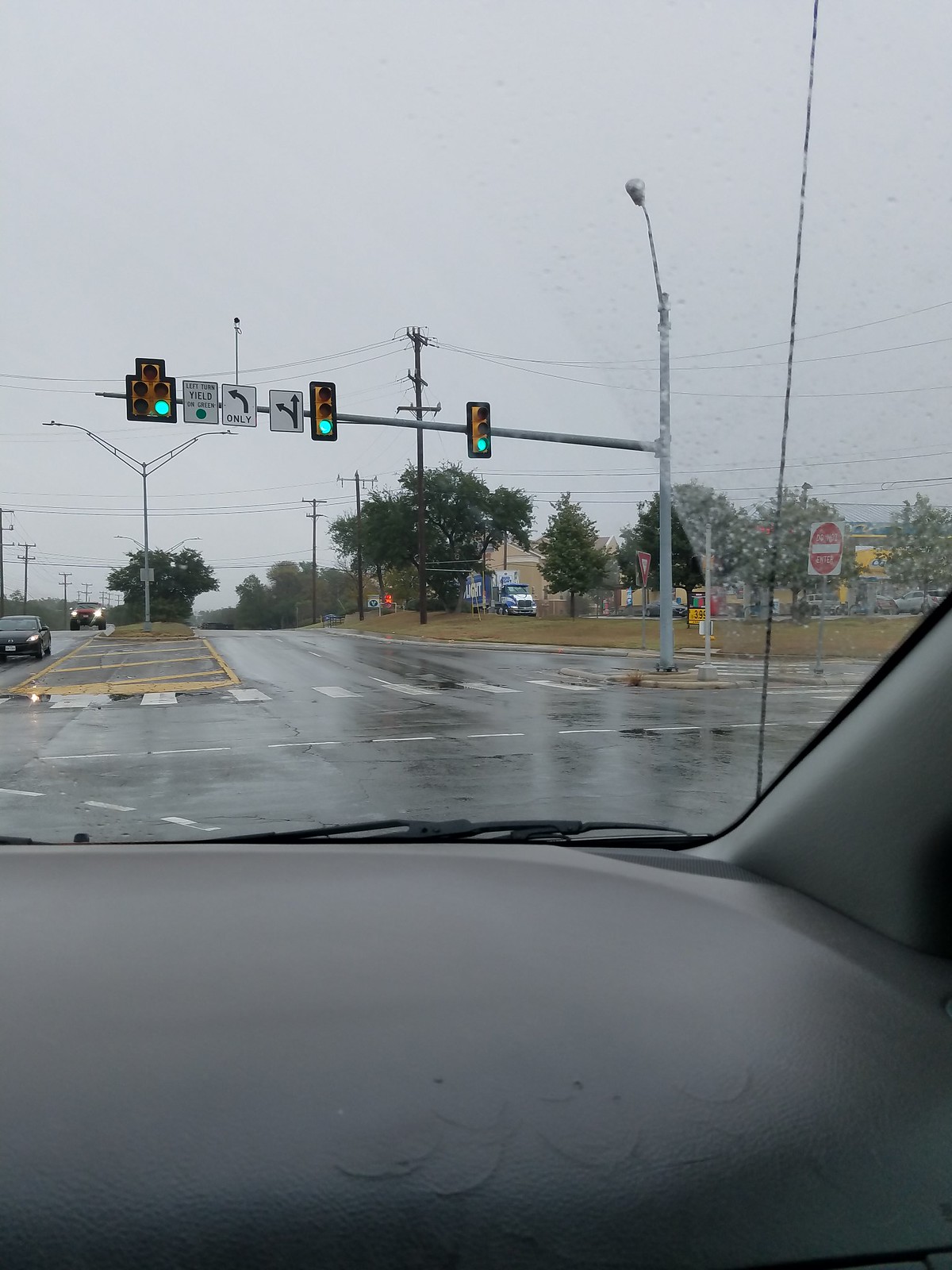View from the right-hand passenger seat of an automobile stopped at an intersection on a rainy day. The traffic light ahead is green, but there is no green arrow, indicating the vehicle is in a left-turn-only lane, waiting for oncoming traffic to clear before making the turn. The wet pavement shines under the overcast sky, hinting at recent rainfall. Ahead, a crosswalk stretches across the far side of the intersection, leading to a concrete median dividing the boulevard. The road comprises two lanes on either side, separated by the median. Across the intersection to the right, a small shopping center with a parking lot and scattered trees is visible.